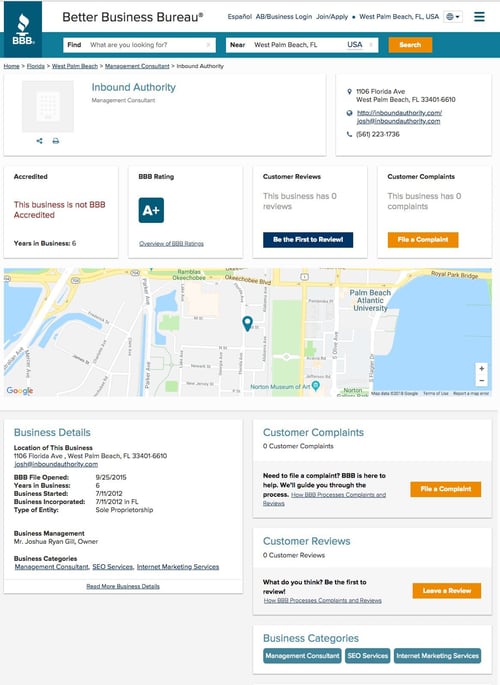This image is a screenshot from the Better Business Bureau (BBB) website. On the left side, the BBB's logo is prominently displayed; it features a white flame reminiscent of the Olympic flame, set against a greenish-blue background. To the right of the logo, the acronym "BBB" is written in white. Above all this, "Better Business Bureau" appears in bold black text. 

In the middle section of the screenshot, there is a "Find" search bar and an "Address" bar labeled "Near," which includes the location information. An orange search button with "Search" written in white is positioned beside these bars.

Below the search function, there is a section marked by a tab titled "Inbound Authority." This section lists the business address as 1106 Florida Avenue, West Palm Beach, Florida, along with a contact number, which appears to be (561) 223-1736.

Further down, there's information about the business's BBB status. The business has an A-plus rating but is not BBB accredited. There are no customer reviews and no customer complaints listed. Below this information, a Google Map displays the business location again as 1106 Florida Avenue, West Palm Beach, Florida. As emphasized, there have been no complaints or reviews for this business.